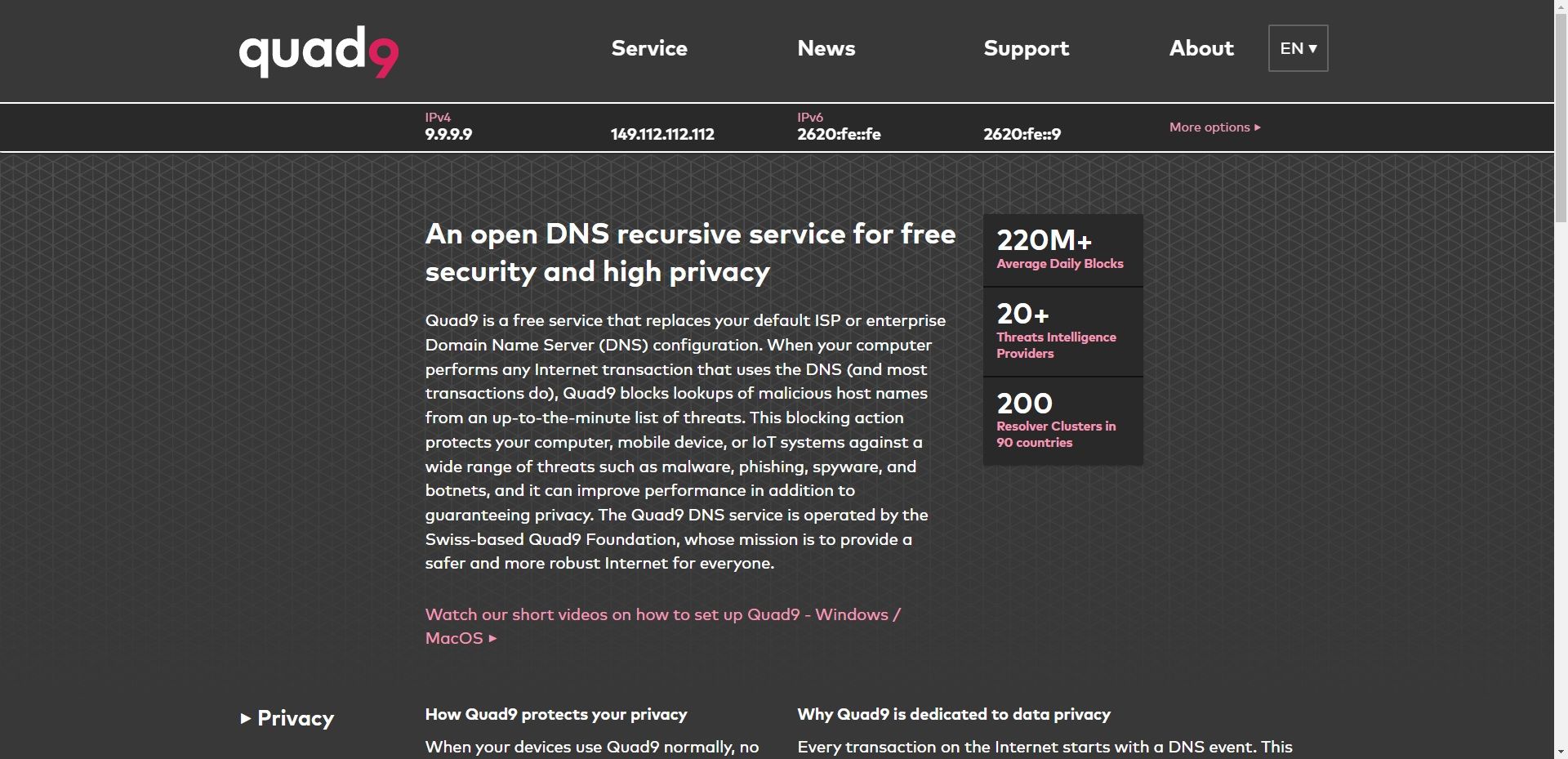This image showcases the official website for Quad9. The top section of the website features a predominantly black background with the word "quad9" in white lowercase letters, where the numeral "9" is in red. The design creatively aligns the top part of the "9" with the lower part of the "d" and extends downward to the end of the "q". 

Below this title, the navigation menu includes options such as "Service," "News," "Support," and "About." Additionally, there is an "EN" button enclosed in a small box for language selection, suggesting a dropdown menu for more language options.

The main content area is framed by a white box, presenting various options related to IPv4 addresses. The key addresses listed are "9.9.9.9" and "149.112.112.112," among others. A link labeled "More Options" in red provides further details.

Dominating the central part of the screen is a large white box with a subtle crisscross pattern in the background. This section highlights Quad9's main service offering with the text: "An Open DNS Recursive Service for Free Security and High Privacy." Adjacent to this, a black box offers impressive statistics including "220 million plus average daily blocks," "20 plus threat intelligence providers," and "200 resolver clusters in 90 countries."

Additional information and resources are provided, including a prompt to "watch our short video on how to set up Quad9" for Windows and Mac users. At the bottom of the page, a "Privacy" button offers insights into how Quad9 protects user privacy and explains why Quad9 is dedicated to data privacy.